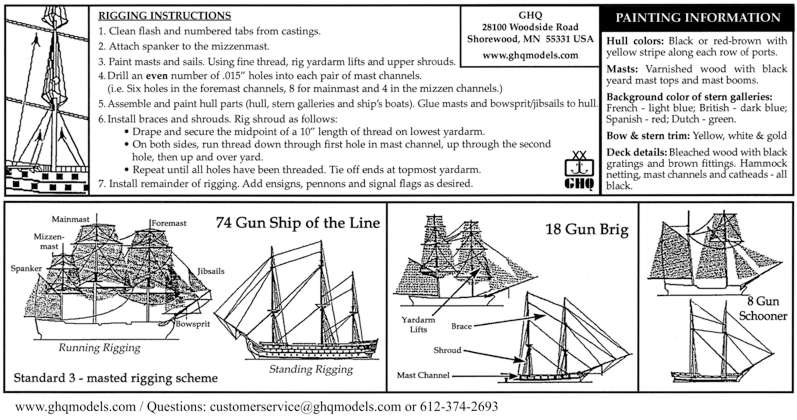The image is a detailed, black and white instructional diagram for building and rigging model ships, including an 18-gun brig, a 74-gun ship of the line, and an 8-gun schooner. The layout is divided into several sections, each meticulously outlining the step-by-step process from start to finish. The instructions begin with cleaning flash and numbered tabs from castings and proceed through various rigging tasks, such as attaching the spanker to the mizzen mast, painting masts and sails, drilling 0.015-inch holes in the mast channels, and installing braces, shrouds, and the remaining rigging. Detailed painting instructions cover hull colors, mast, stern galleries, bow, and stern trim, and deck details. The diagram, produced by GHQ in Shorewood, Minnesota, also features small, intricate illustrations of the different ship types and their rigging arrangements, with accompanying text for each step, emphasizing precision and accuracy in assembly and painting. The overall presentation is clean, with clear, numbered instructions and fine line drawings that guide the modeler through the entire process.